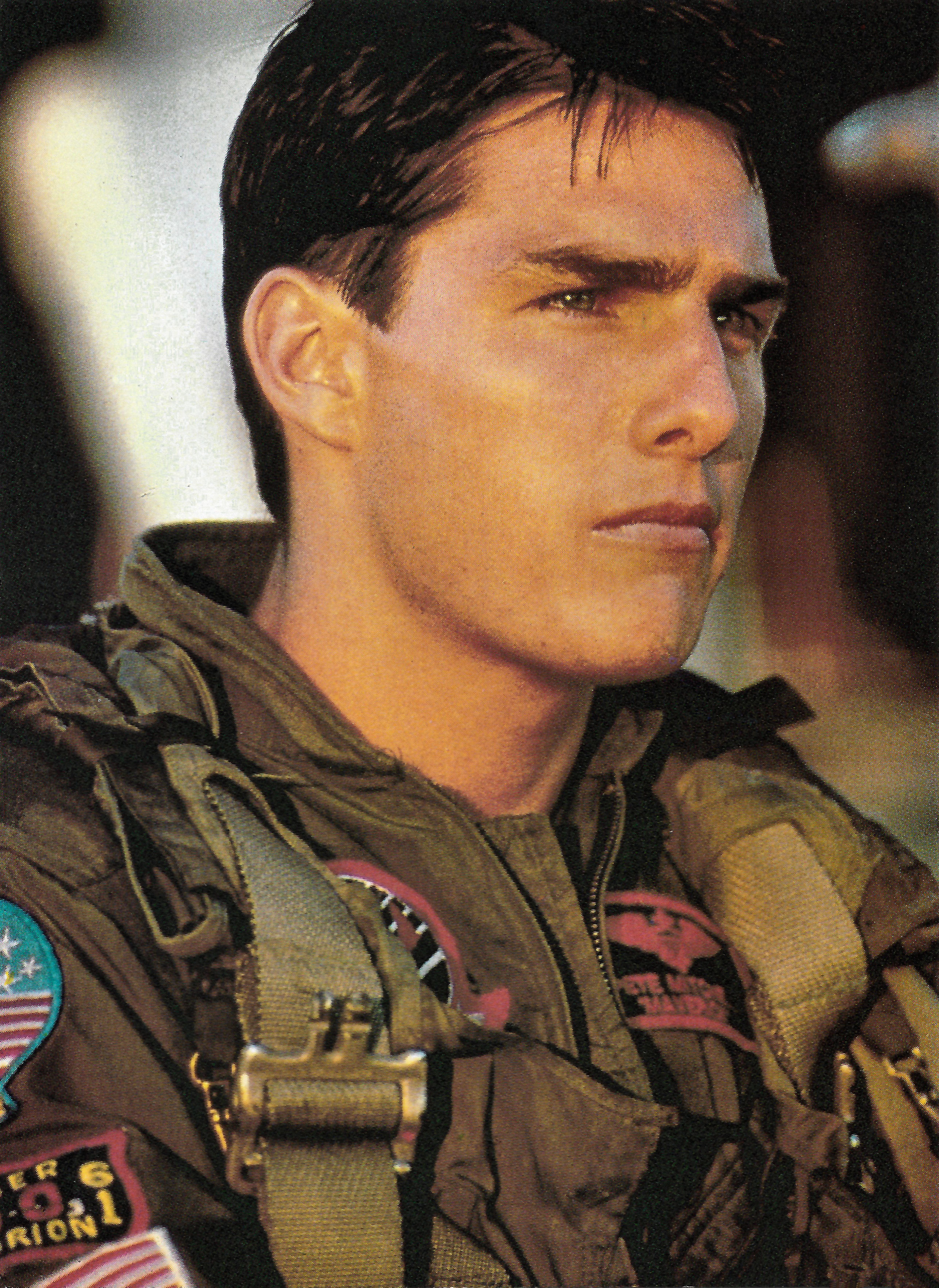This photo captures a young Tom Cruise, likely in his early 30s, dressed in a military aviator uniform from the iconic 1980s movie "Top Gun." The olive-green jumpsuit with tan straps is adorned with numerous insignia and embroidered patches, including American flags on his right arm, one next to a patch that reads "E-R-O-R-I-O-N, 61" in yellow letters on a black background and a red zero, and an eagle patch on his chest. His dark brown hair is closely cropped, with a few strands falling onto his forehead, and he has expressive, downturned eyebrows over light-colored eyes, accentuating his intense, frowning expression. The background is deeply blurred, displaying indistinct patches of red, black, white, beige, and brown hues, creating a focus entirely on Cruise's determined and resolute visage.